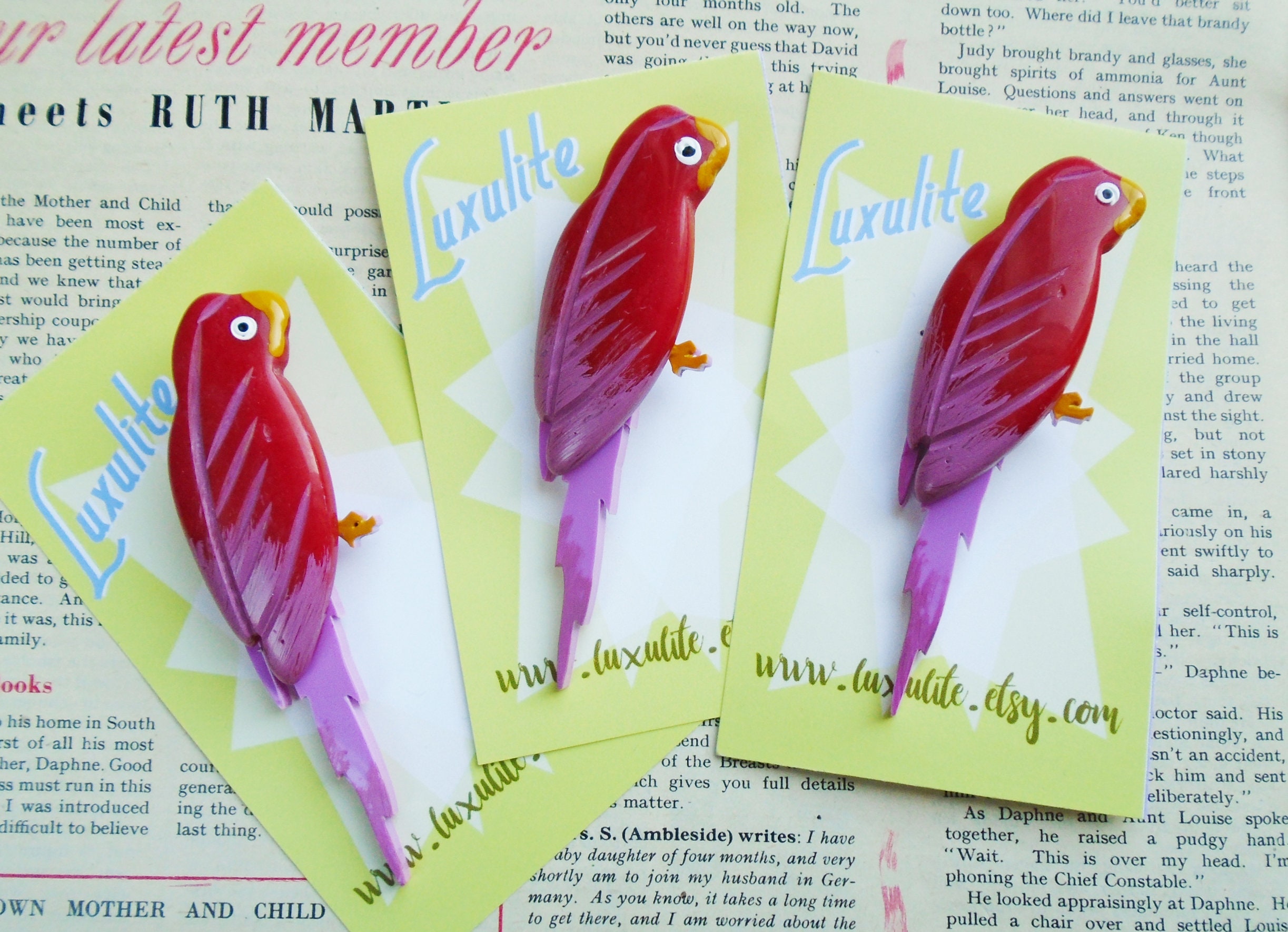This photograph showcases three identical cards arranged in an arc, resembling a spread hand of playing cards, on top of a faded white paper background that appears to be a book or a newspaper. The visible text in the upper left corner of the paper is printed in italicized pink cursive and reads "Latest Member." The cards, each with a lime green background, feature a white starburst design and pale blue text in the top left corner that reads "Luxulite, L-U-X-U-L-I-T-E." Each card displays a three-dimensional cartoon parrot facing away from the viewer. The parrot, made of plastic, has a red body, pink wingtips, and a pinkish-purple tail, with an orange beak and talons. Its eye is a simple white shape with a black dot in the center. At the bottom of each card, in dark green text, is the website link "www.luxulite.etsy.com." The cards likely serve as backing for the pins, which are designed to help sell them in stores or online platforms like Etsy.